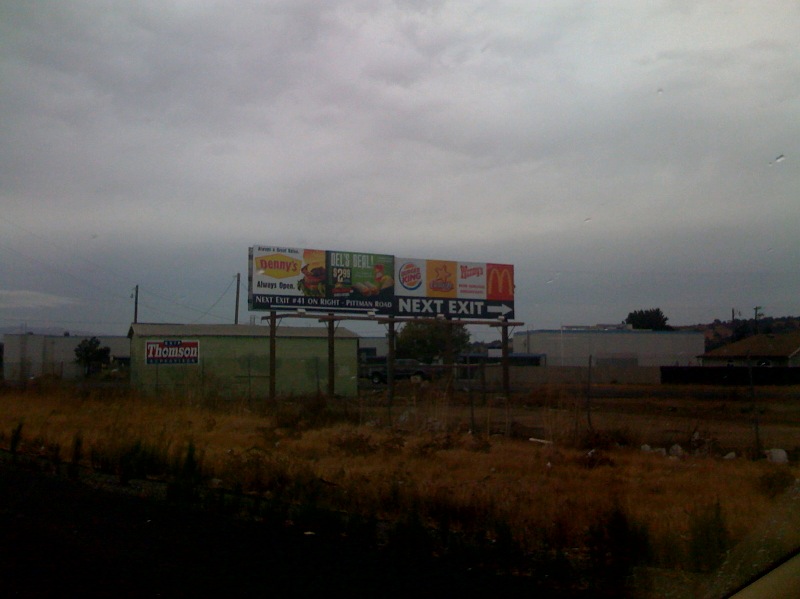In this dimly lit photograph, captured possibly from a car window on a cloudy, overcast day, the primary focus is a pair of adjacent highway billboards framed against a backdrop of industrial buildings. The scene appears to be during early spring or late fall, as the vegetation is a brownish color, not yet green. The first billboard prominently advertises Denny's always-open service with an enticing $2.99 breakfast deal labeled "Dell's Deal," instructing travelers that Denny's can be found at the next exit, number 41 on Pittman Road, with an arrow pointing to the right. The second billboard is unique as it simultaneously promotes four fast-food giants—Burger King, Hardee's, Wendy's, and McDonald's—all sharing a singular message directing drivers to the "Next Exit" with another right-pointing arrow. Nearby, one of the industrial buildings has a green sign that reads "Thompson," while the others appear nondescript. The overall ambiance is dark and grey, contributing to a somewhat somber but highly detailed roadside scene.